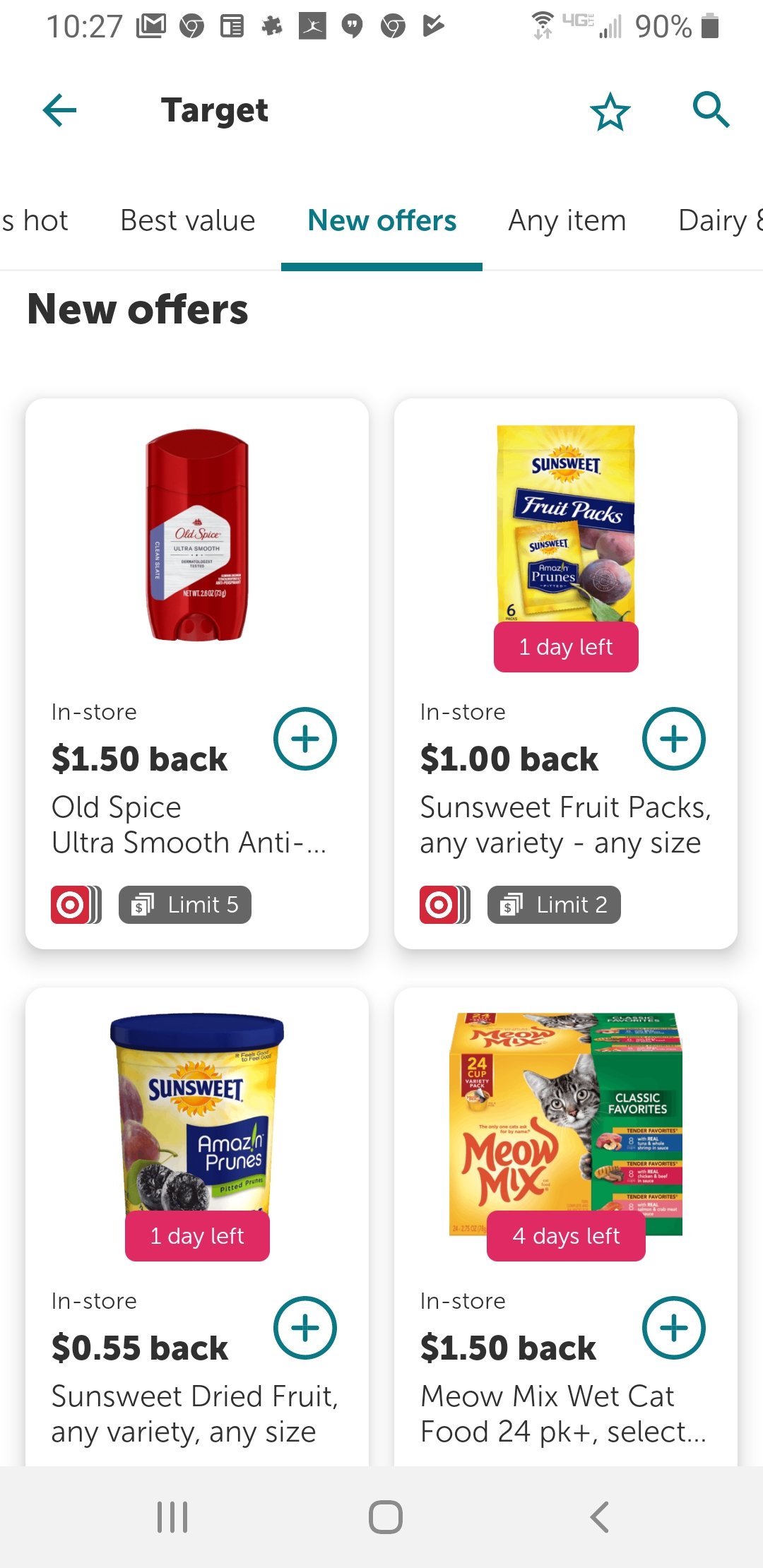Here's a detailed and cleaned-up descriptive caption based on the provided voice description:

---

This rectangular portrait image appears to be a screenshot taken on a smartphone, showcasing various online shopping offers. The background is predominantly white, without any borders. At the very top, the status bar displays the time as 10:27, followed by a series of seven icons. These icons include a dark rectangle with the letter 'M,' a gray and white version of the Google Chrome icon, a battery indicator showing 90% charge, and a nearly full vertical battery icon in the top-right corner.

Below the status bar, on the left, a blue arrow points to the left. Next to it, the word "Target" is written in black. On the far right, there is an empty blue star and a blue magnifying glass icon for search functionality.

A row of text menus follows, starting with a partially visible menu ("Hot" and "s hot"), followed by clearly visible options: "Best Value," "New Offers" (highlighted in bold teal with an underline), "Any Item," and a cut-off option labeled "Dairy."

The main portion of the image is divided into four sections showcasing product images and corresponding offers:
- **Upper left**: An Old Spice red canister, priced with a rebate of $1.50.
- **Upper right**: A package of SunSweet fruit packs with $1.00 back.
- **Lower left**: A canister of SunSweet Amaz!n Prunes, offering $0.55 back.
- **Lower right**: A large box of Meow Mix 24-pack wet cat food, offering $1.50 back. 

Each product listing includes descriptive text beneath the image, such as "Meow Mix, wet cat food 24 pk plus select..." The lower right of each product listing features a green circle with a green plus sign.

Lastly, a thick light gray navigation bar extends across the bottom, featuring three icons: three vertical parallel bars on the left, a square with rounded corners in the middle, and an arrowhead pointing left on the right.